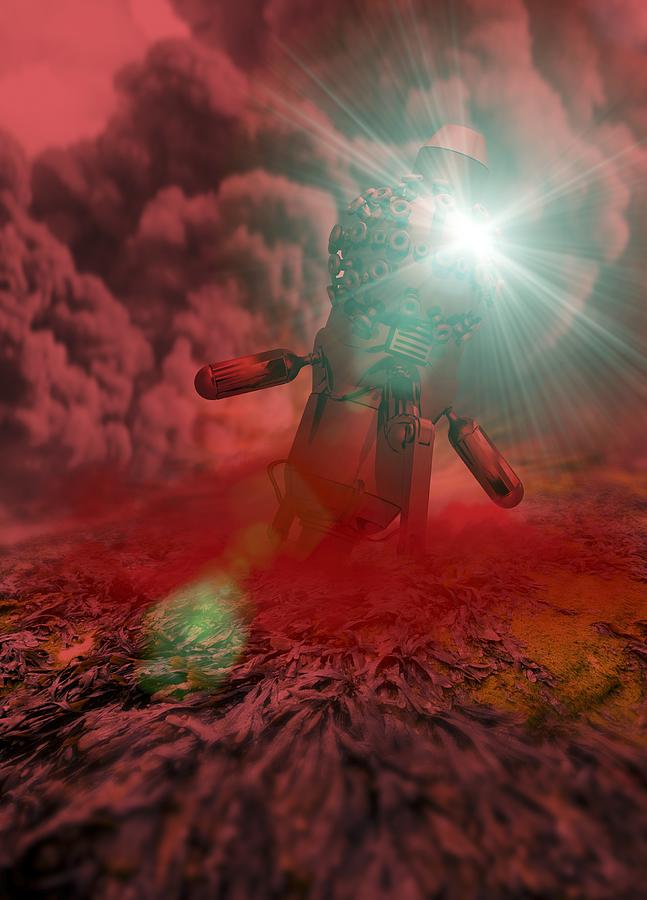This digital art image features a central robot with a round, multi-holed head emitting bright, blinding white light from one of the holes. The robot's cylindrical hands and metallic body are painted red. It stands on a ground scattered with dry leaves or bark in shades of red, yellow, and brown. Behind the robot, a large cloud of gray smoke merges with a burst of red smoke at the top, encasing the scene in a smoky, red filter. The textured foreground displays a mix of reddish, orange, purplish, and black hues, adding depth and contrast to the overall composition.